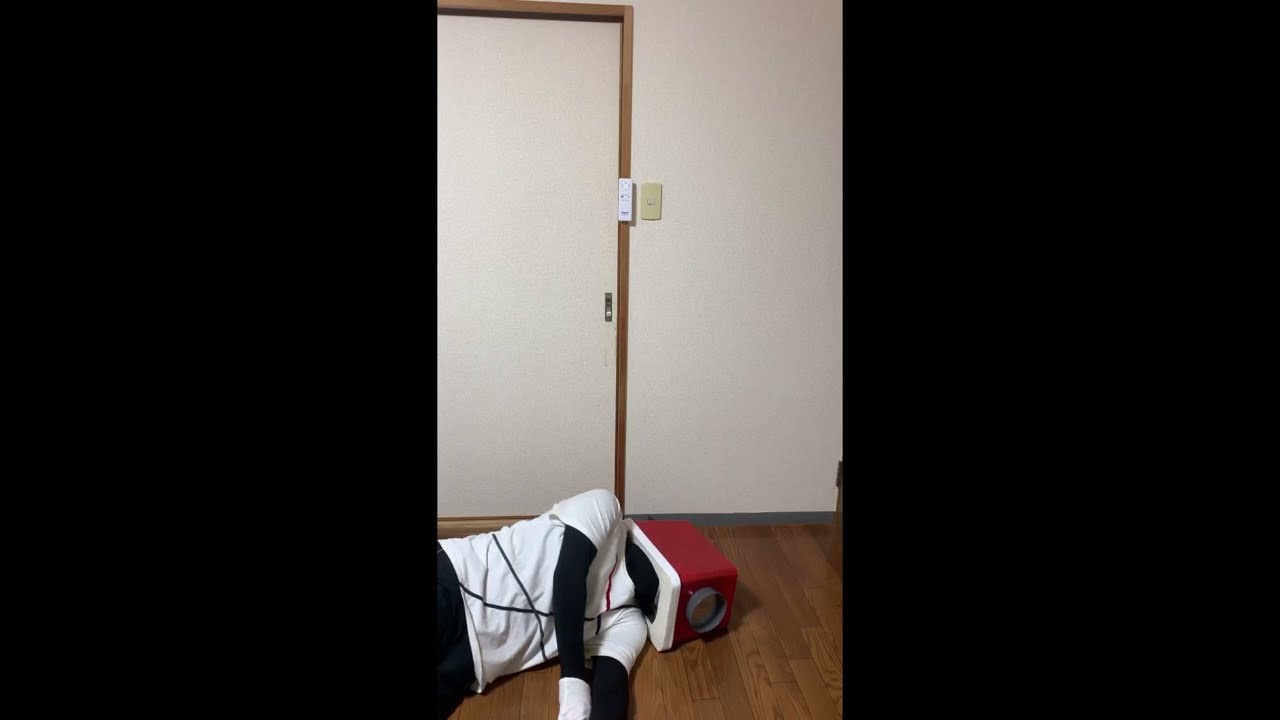In this photograph taken inside a room, a person is lying on their left shoulder on a brown hardwood floor. The person is dressed in a long-sleeved black shirt beneath a white t-shirt adorned with black and red stripes, black pants, and white linen gloves. Covering their head is a distinctive maroon rectangular box with an off-white base; the box has a small plastic lens or round window on one side, suggesting a performative art piece. The backdrop features a white door with a brown wooden frame on the left side of the image and another white door at the back. Additionally, there are two switches: one white switch on the brown frame and another beige switch on the white wall towards the right. The scene overall suggests an unusual and intriguing tableau.